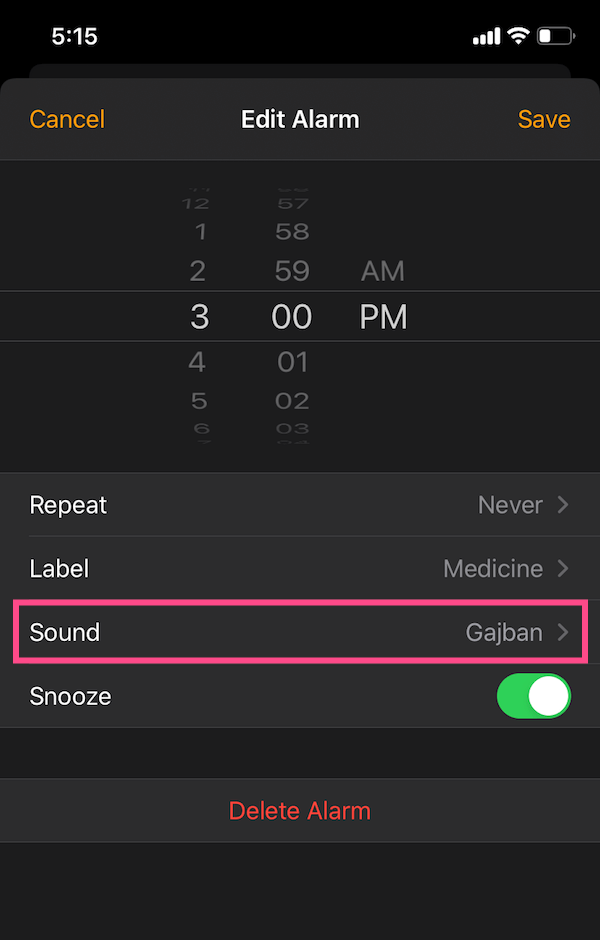This is a detailed screenshot of an iPhone's alarm editing screen set for 3:00 p.m. The interface clearly shows the "Edit Alarm" title at the top, with options to "Cancel" on the left and "Save" on the right, both highlighted in orange. Below the time settings, there are several customizable fields: "Repeat" (currently set to "Never"), "Label" (labeled as "Medicine"), "Sound" (highlighted in pink for emphasis), and "Snooze" (toggled on in green). At the bottom of the screen, there is a "Delete Alarm" button in red. 

Additional iPhone-specific UI elements are visible in the status bar at the top of the screen. On the upper left, the time is displayed as 5:15, while the upper right shows icons for cellular signal strength, Wi-Fi connectivity, and battery level. The unique pink outline around the "Sound" option suggests the user intended to draw attention to the available ringtones or alert sounds for this alarm.